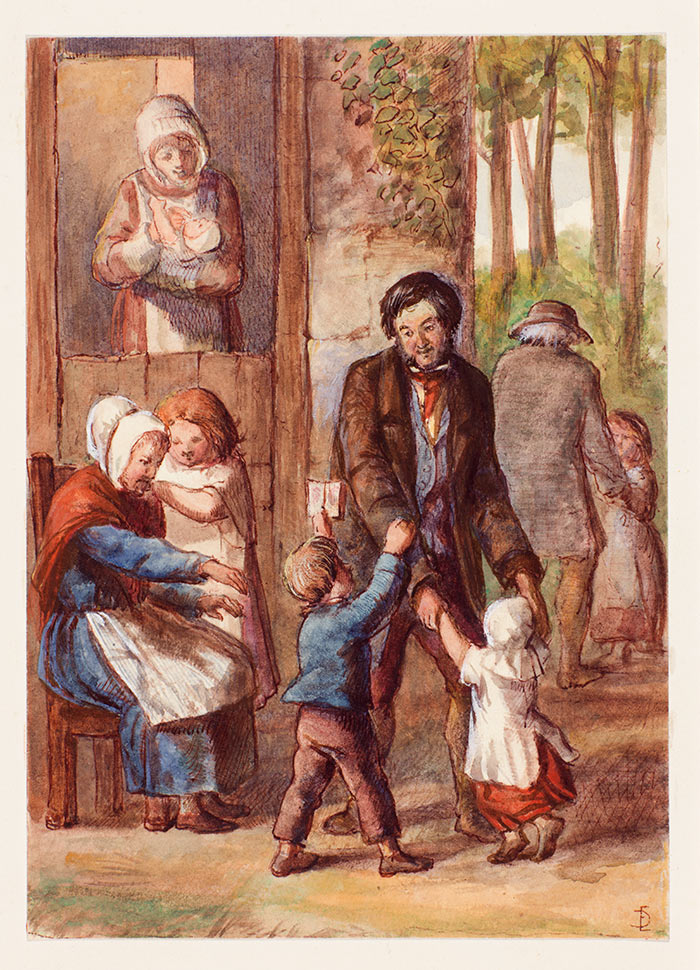This painting, reminiscent of the early 1800s or late 1700s, depicts a lively scene of olden days set against a backdrop of a wooded area and an old structure. Central to the image is a man in a brown suit with a sash-like tie, lovingly looking at a little boy who tugs on his right arm. The boy, facing away, is dressed in a blue long-sleeve suit jacket, long brown pants, and brown shoes. Beside him, a little girl in a white bonnet, white shirt, and red dress holds the man's hands as they dance. An older woman, seated and reaching out to join hands with the boy, wears a bonnet, a blue dress, a white apron, and a red shawl, which is being adjusted by another little girl standing behind her. Occupying the foreground, this group of figures contrasts with other background activities: a woman at a window tenderly attending to a baby, and an older man dancing with another little girl in the mid-right section of the picture. The overall scene captures a harmonious blend of interaction and joy, framed by the natural and architectural elements of the period.